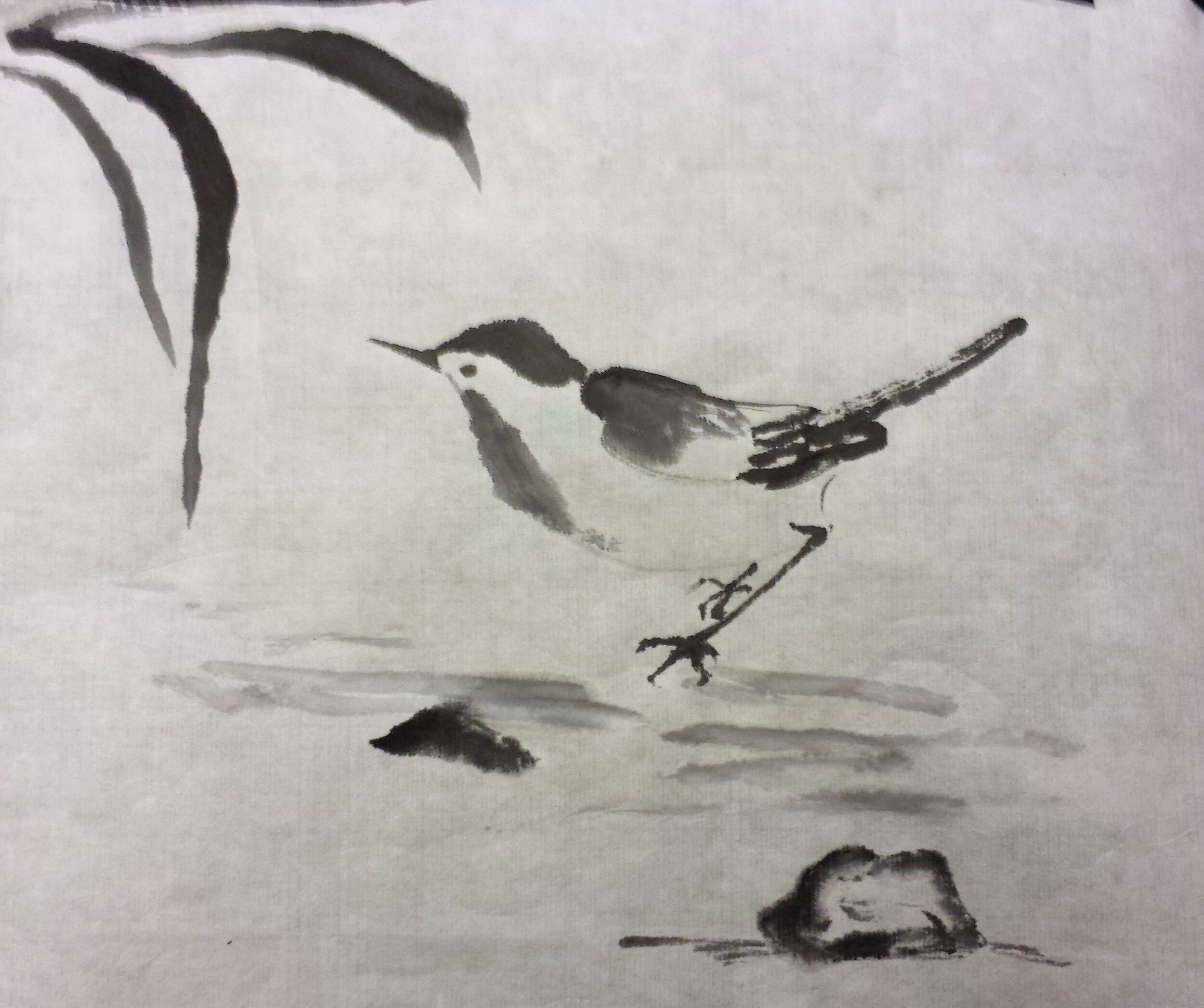This image is a highly detailed grayscale drawing, potentially using watercolor or charcoal, with minimalistic and expressionistic Japanese influences. Set against a light lilac mottled background, the artwork centers on a bird with a long, pointed beak. The bird stands poised on narrow, slender legs and is characterized by a dark head, a dark upper wing section, white mid-wing feathers, a very dark tail with hints of white, and a belly that transitions from gray at the neck to white. To the bird's left, three or four leaves hang, suggesting the presence of an unseen tree or plant. The ground beneath the bird is subtly indicated by a few brush strokes, with two or three small, abstract rocks adding to the scene's simplicity. The entire piece uses only neutral tones, creating a monochromatic yet evocative representation.